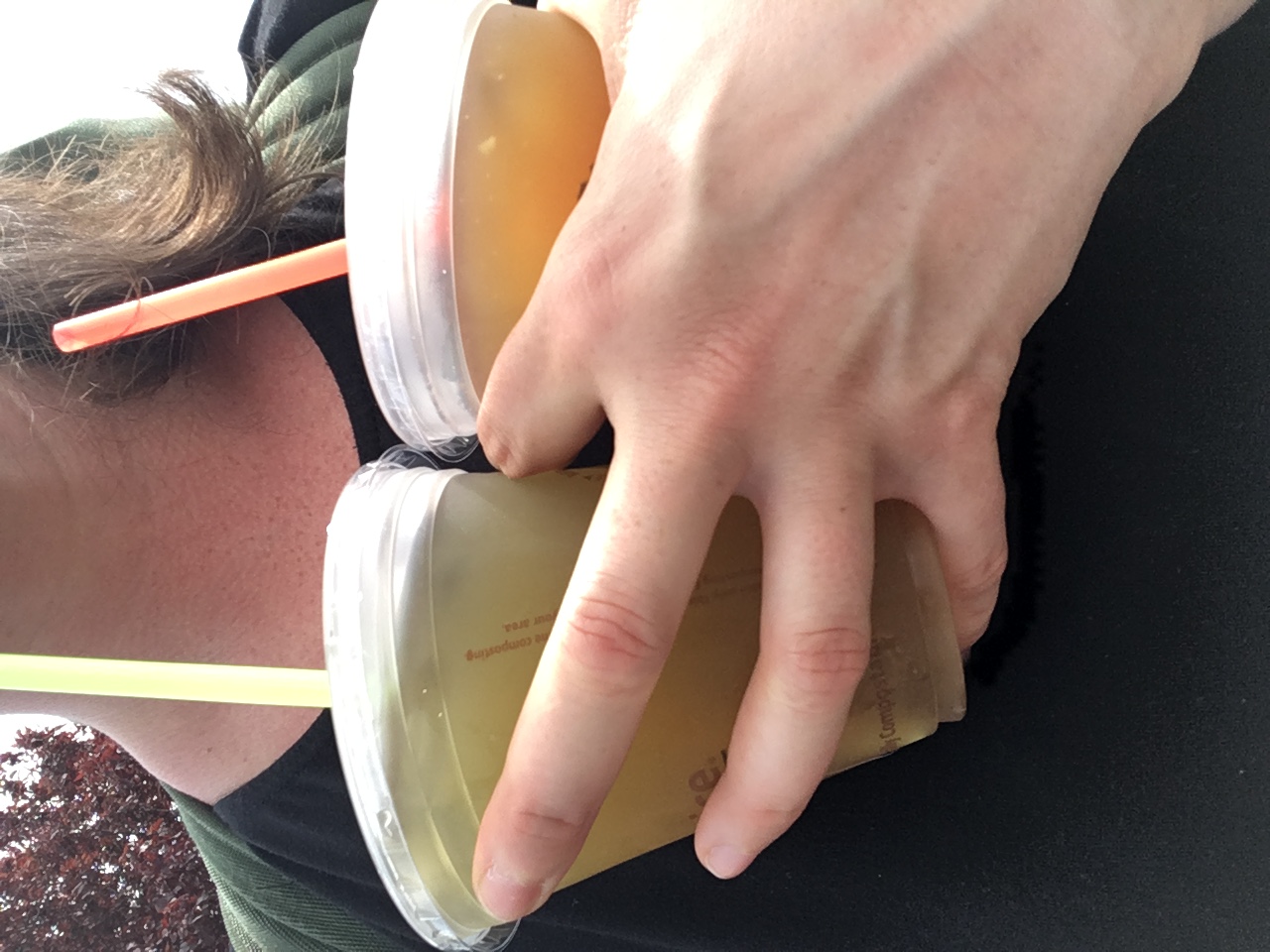In this outdoor scene, a woman with light-colored skin and shoulder-length brown hair is holding two clear plastic cups with clear lids tightly against her chest, using one hand. Her face is not visible; the image captures her from the neck down, showcasing a green shirt with a rounded neckline. The drink in her hand by her thumb contains a brownish liquid and has an orange straw, while the drink held by her middle fingers contains a greenish liquid with a light green straw. Behind her, the sky appears dreary, and a tree with reddish-brown leaves is visible in the top left corner of the image.